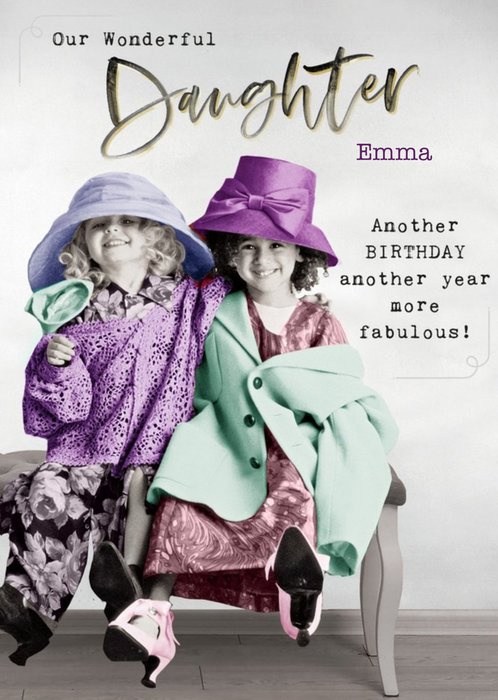The image features a charming birthday card showcasing two young girls dressed in oversized, playful attire, reminiscent of dress-up from their mom or grandma's wardrobe. The card celebrates "our wonderful daughter Emma," with the text elegantly displayed in a combination of gold and black fonts, and Emma's name highlighted in purple. 

The room they're in has a gray wooden floor and a matching gray wall as a backdrop. Both girls have curly hair and wear infectious smiles. The girl on the left has blonde curls and is donned in a black dress adorned with purple flowers, topped with a purple sweater that has holes, and a large blue hat. She's also wearing oversized shoes. The girl on the right, with dark, tight curls, sports a purple dress with swirls, a white shirt underneath, and a green trench coat draped over her shoulders. She accessorizes with a large purple hat featuring a big bow and pink high-heeled shoes. They sit closely on a bench with their arms wrapped around each other, embodying the joy and whimsy of childhood play. The card concludes with the phrase "another birthday, another year more fabulous," celebrating Emma's special day with a touch of loving humor.